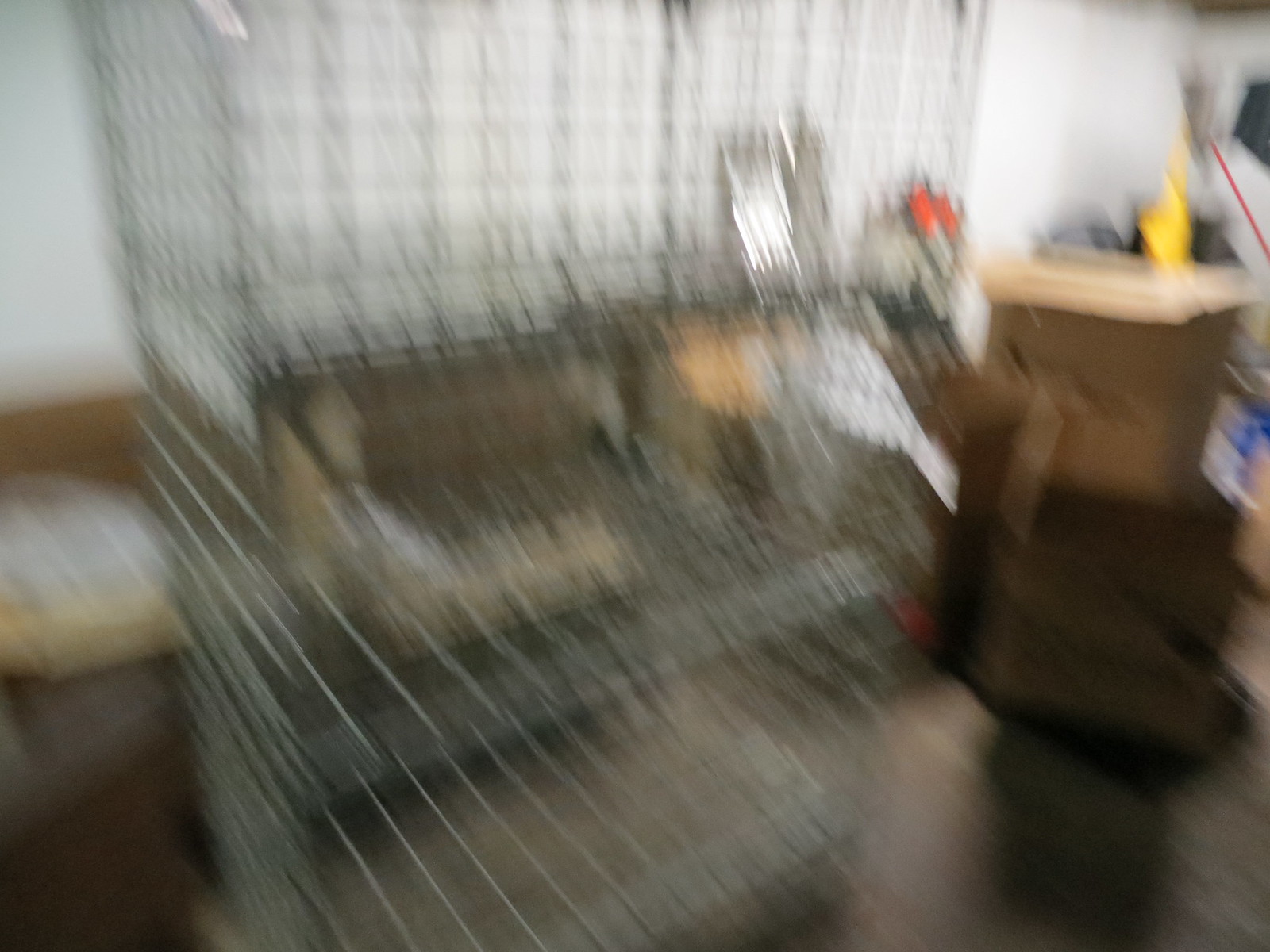A blurry image captures the interior of a room dominated by a large rectangular metal cage situated at its center. In the back left corner of the room, a couch is faintly discernible, suggesting a casual seating area. The back right corner features an array of stacked boxes, adding an element of disorganization. The walls vary in appearance: the back left wall is stark white, while the back right wall incorporates metallic elements. Some indistinct yellow items are scattered in the background, adding a splash of color. The floor, which has a brown hue, complements the room's overall utilitarian aesthetic. The image suffers from motion blur, further obscuring the scene and making it challenging to discern specific details, particularly amidst the clutter in the back right.